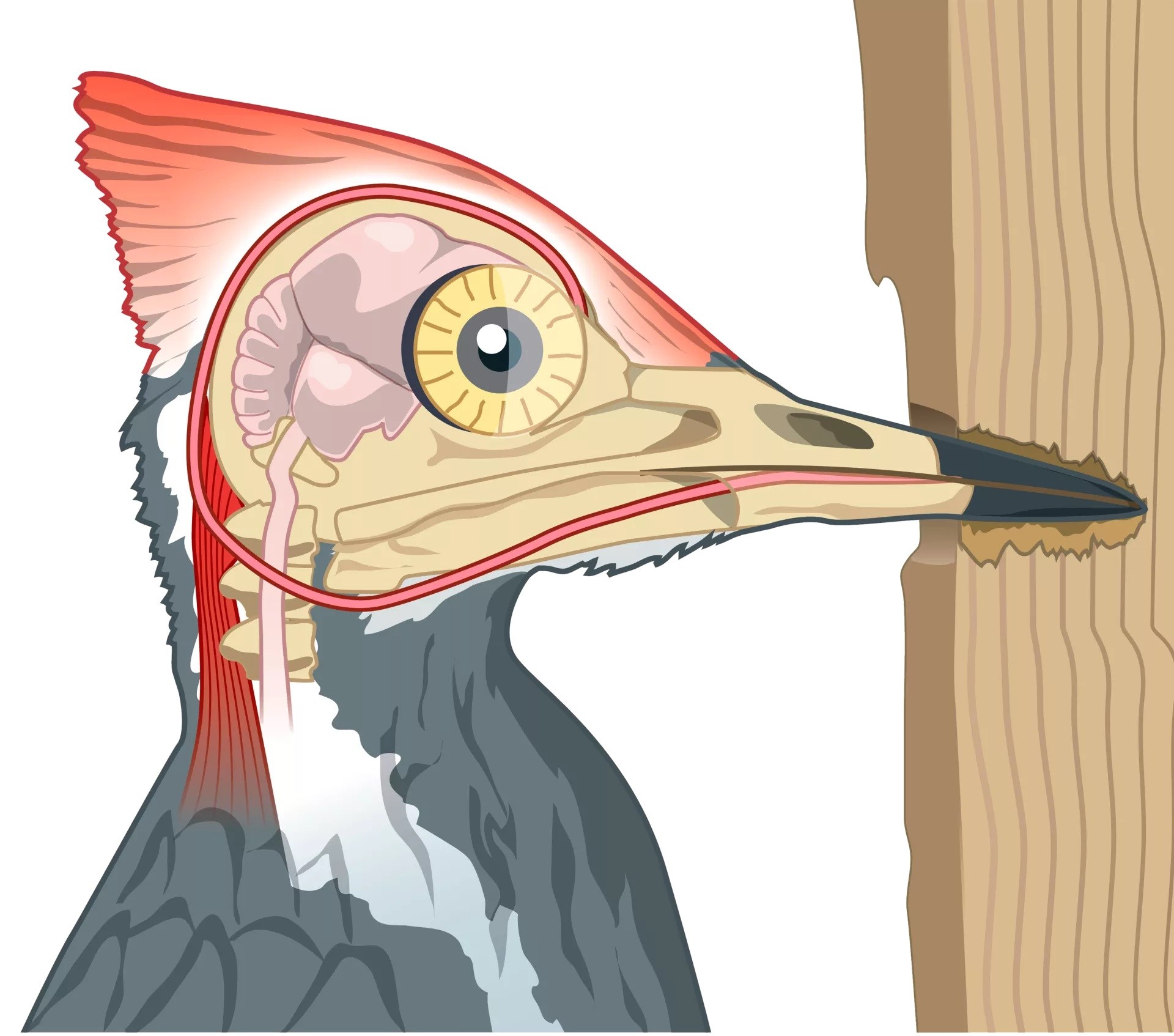The image features a detailed cartoon illustration of a woodpecker set against a white background. The woodpecker is depicted in a cross-sectional view, facing the right side of the picture, where its black-tipped beak is embedded into a piece of vertical-grain brown wood. This cross-section reveals the inner anatomy of the bird, including a brain and a spinal cord highlighted in light pink, as well as muscles in the back of its red head. The bird's eye, which appears prominently large and wide open, is yellow with a black center featuring a white dot, indicating a serious or surprised expression. The body of the woodpecker is gray with subtle white shadings, and additional details show the beak working to gnaw out wood, emphasizing the bird's characteristic pecking behavior.